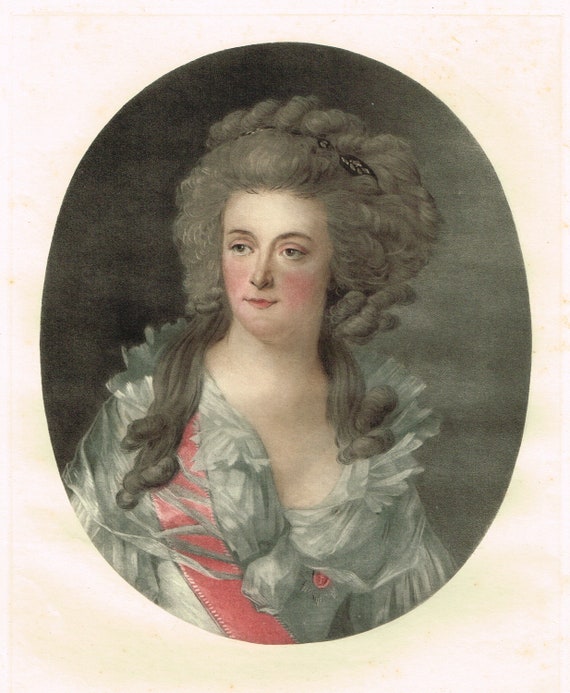This meticulously detailed image depicts a portrait of a woman from what appears to be the 19th century. The composition is arranged within a vertically oriented, rectangular frame with a distressed, cream-colored background accented with hints of white and yellow highlights. At the center of this background lies an oval-shaped, gray vignette that frames the woman's likeness.

The woman sports a dramatic coiffure with voluminous gray hair piled high on her head, complemented by a black scarf or headband interwoven with the hair. Her curly hair cascades in long spirals down to her shoulders and chest, with some curls hanging freely at the sides. Despite the possibility of the hair's texture differing from its extensions, it presents an overall uniformity in its grand appearance.

Her complexion is very light, almost pale, with distinctively rosy pink cheeks that enhance her refined, yet soft expression. She gazes outward in a subtle diagonal direction to her left, with her thin lips forming a gentle, nearly imperceptible smile. The woman wears a striking dress, predominantly gray with white accents and characterized by elaborate lace ruffles adorning the neckline and shoulders. The dress features billowy sleeves and a corseted bodice, further emphasized by a distinguishing red sash draped from her left shoulder (as observed in the frame) to her right, secured with a red button. The entire portrait is encased in a subtle black border, giving it a historical and elegant finish.